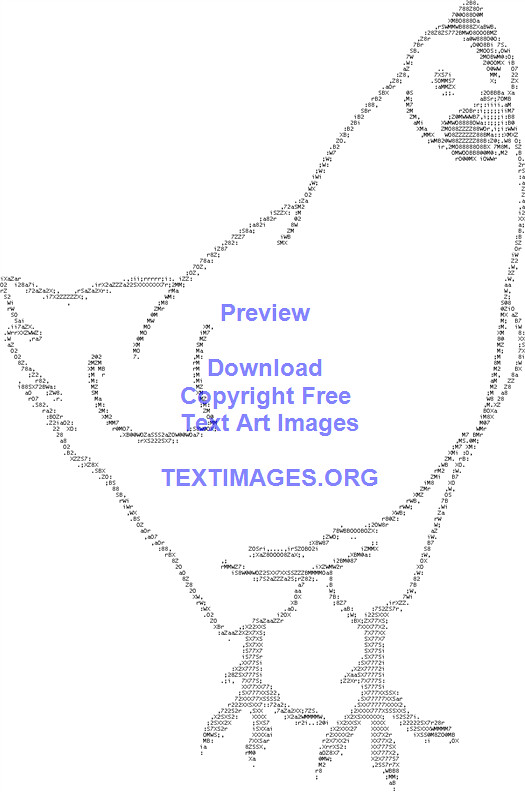This is an illustrated, text-art image of a chicken created using a series of numbers or dots against a plain white background. The image appears to be a black-and-white outline of a chicken standing on its two feet, facing forward and slightly to the right. The chicken's silhouette is detailed enough to distinguish features like feathers on the left, a tuft on its head, its beak, and its right eye. In the middle of the chicken, there is blue text that reads "preview, download, copyright free, text art images, textimages.org." The text art, also referred to as ASCII art, cleverly uses these characters to form a recognizable image with an abstract touch. This combination of digital craft and minimalistic design makes the chicken's depiction both accurate and intriguing.